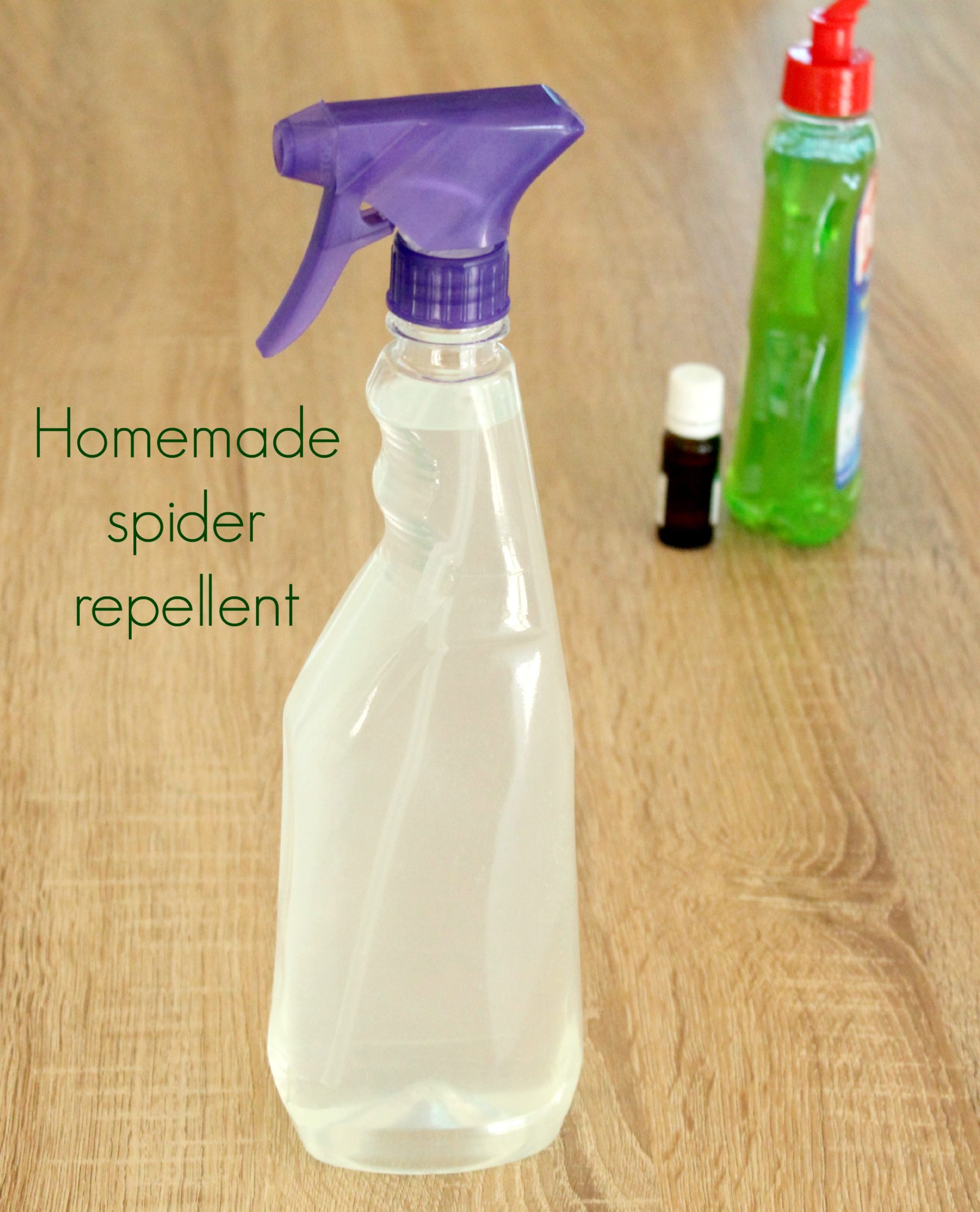In this image, three distinct bottles are placed on a light wooden table. The most prominent bottle, situated slightly to the left in the foreground, is a large clear plastic spray bottle with a purple screw-on spray top. It is filled nearly to the top with a cloudy, whitish liquid, and on the left side of the bottle, green text reads "Homemade Spider Repellent." 

Behind this spray bottle, in the background to the right, stands a green soap bottle with a red pump-action lid. The label on this bottle is turned to the side and is not clearly readable, but it appears to be a dish detergent.

To the left of the green soap bottle, there is a much smaller brown vial, roughly an inch tall. This tiny bottle, which resembles an essential oil container, has a white twist-off cap. The bottles in the background are slightly out of focus, emphasizing the clear spray bottle in the front.